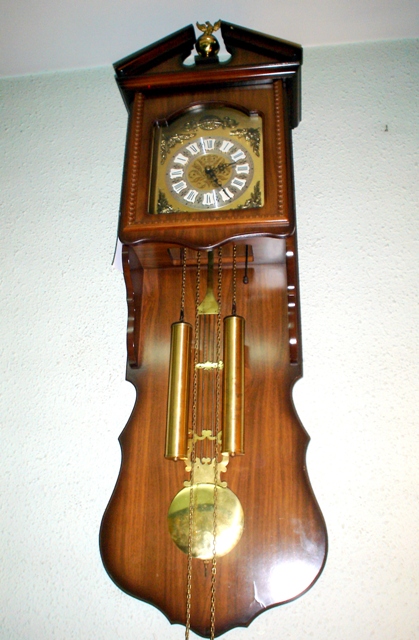This beautifully crafted wooden wall clock is a nostalgic, pendulum-style timepiece reminiscent of those commonly found in grandparents' homes. The clock features a distinct house-shaped top, crowned with an intricate gold figure of a bird perched on a globe. The clock face itself is a radiant gold color, adorned with clear white numbers and ornate hands. Below the clock face, long chains extend from the weights and pendulum, set against a protective wood panel. The wood paneling is elegantly shaped, resembling the curvy outline of a violin. This classic clock, mounted on a pristine white wall, exudes timeless elegance and charm.